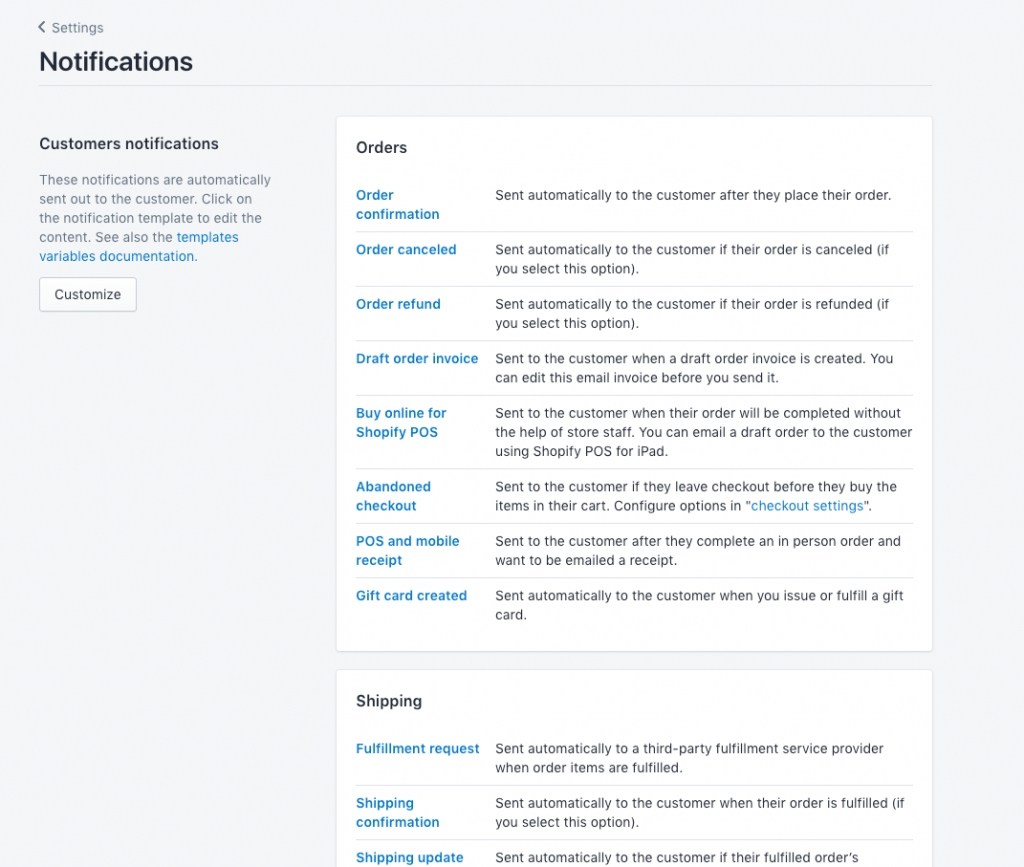The image depicts a web page on a computer with a very light grey background. The web page follows a square orientation and is dedicated to user notifications. At the top left corner, there is a navigational element labeled "Settings" with a left-pointing arrow beside it. Below this label, the heading "Notifications" is prominently displayed. A brief instructional paragraph explains that customer notifications are automatically sent out to the customer and advises users to click on the notification template to edit its content. Additionally, it mentions the availability of template variables documentation for further customization. Beneath this paragraph, there's a "Customize" button for users to tailor their notifications.

On the right side of the page, there are two distinct sections. The first section is enclosed in a square box labeled "Orders." Under this heading, a column lists categories in blue text: "Order Confirmation," "Order Cancel," "Order Refund," "Draft Order Invoice," "Buy Online for Shopify POS," "Abandoned Checkout," "POS and Mobile Receipt," and "Gift Card Created." Each category is accompanied by explanatory text to its right, detailing the specifics of each notification type. The second section, positioned below and partially cut off at the bottom of the image, is a horizontally rectangular box labeled "Shipping." This section includes categories such as "Fulfillment Request," "Shipping Confirmation," and "Shipping Update."